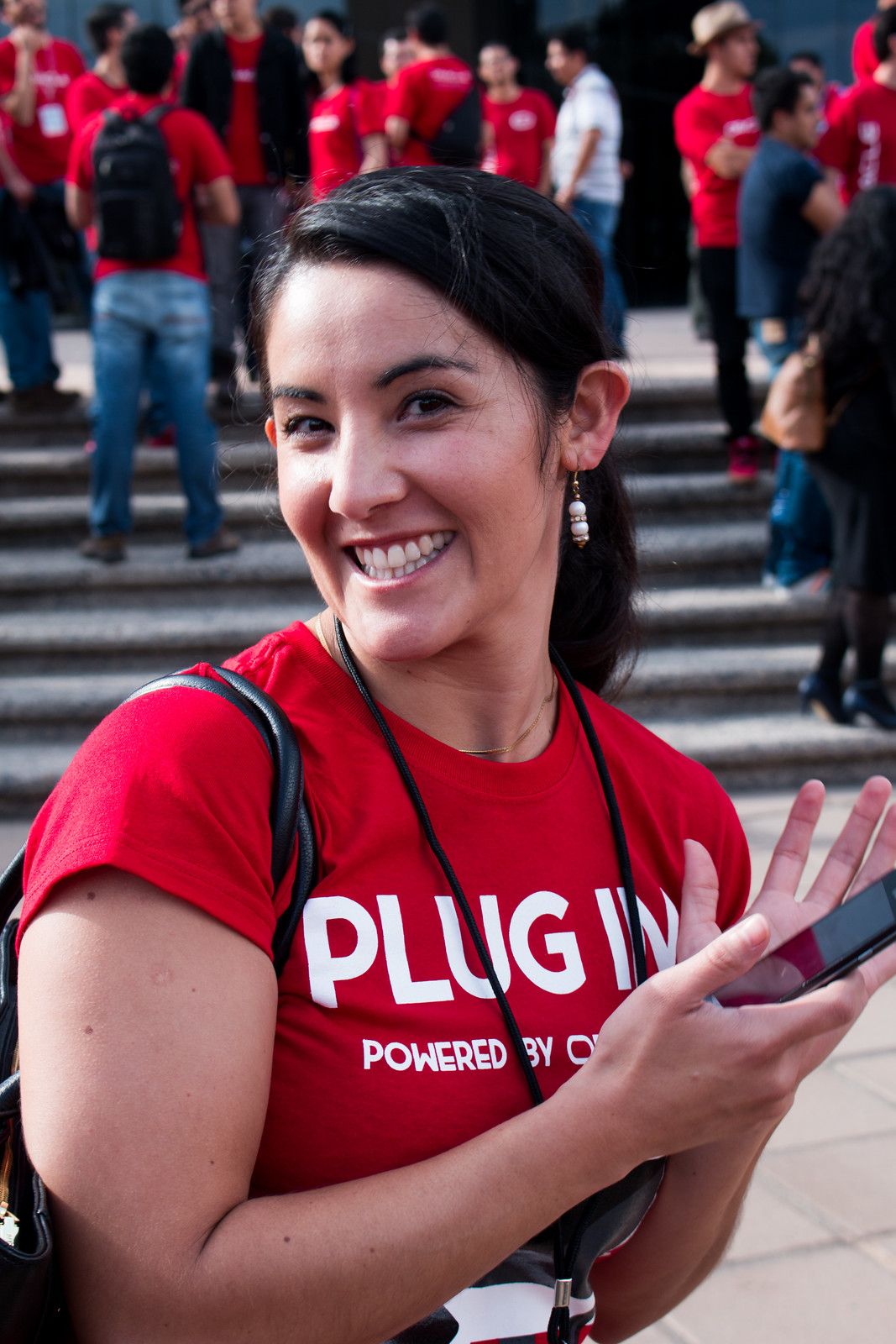In this photograph, a woman with dark hair pulled into a low ponytail stands at the center, smiling broadly at the camera. She's wearing a red short-sleeve crewneck t-shirt with white text across the front that reads "Plug-in" followed by "powered by." A black lanyard and a tight necklace hang around her neck, and a strap from her purse is draped over her left shoulder. She's holding a black smartphone in both hands at chest level, partially obscuring the text on her t-shirt. Her white earrings add a subtle contrast to her dark hair. Behind her, a group of people, all wearing similar red t-shirts and jeans, are gathered on gray cement steps. One man stands out in a white t-shirt. The background is slightly out of focus, emphasizing the group's gathering while indicating a possible student event. The steps and the tiled ground contrast with the vibrant red of the t-shirts, enhancing the overall composition of the image.